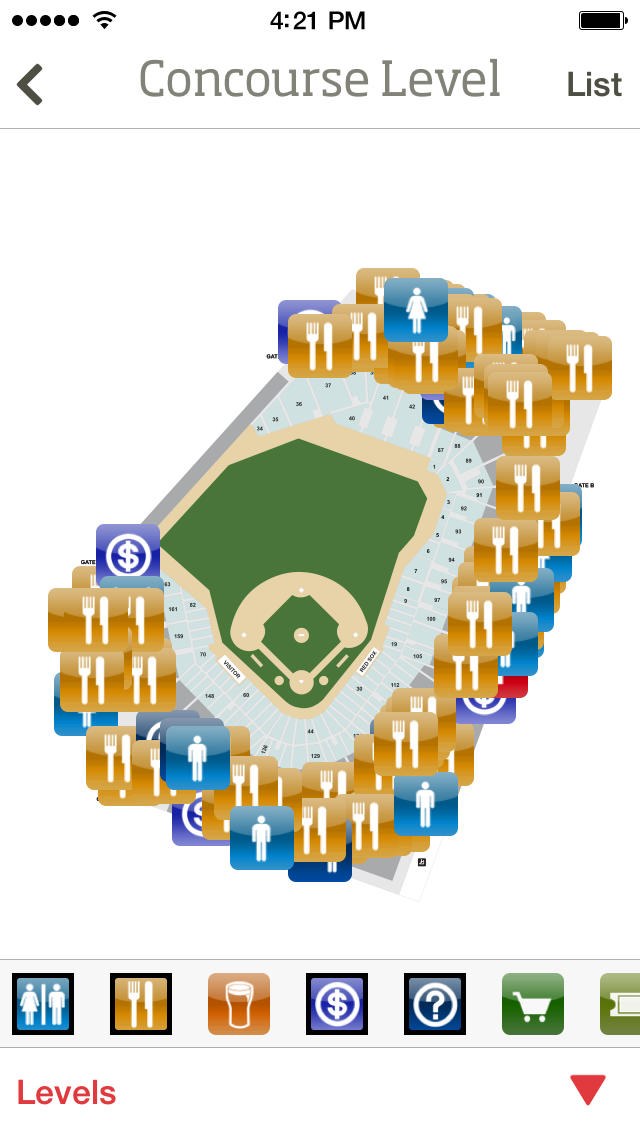The image appears to be a screenshot from a mobile phone, capturing a digital map or app interface, designed for navigating a stadium. The top part of the image shows a header with the time "4:21 PM" displayed, and an icon indicating a fully charged battery. Below this, there is a faint gray line, next to which the word "List" is faintly visible. The central portion of the image features a digital illustration of a baseball diamond, colored in green with beige areas marking the bases, although it’s relatively small and schematic.

Surrounding the baseball diamond are various icons indicating the amenities within the stadium. Numerous knife-and-fork symbols indicate the locations of eating areas, while blue icons depicting standing figures suggest the locations of restrooms. Additional icons, including money symbols and burgundy icons, are also scattered around the area, providing further navigation cues.

At the bottom of the image, there is a strip containing a row of icons denoting essential services, such as restrooms, food and drink stations, cash points, information services (indicated by a question mark), and carts. There is also a red "Levels" label with a down-pointing arrow, possibly indicating the option to switch between different levels or sections of the stadium. 

To the upper part of this interface, "Concourse Level" is displayed with arrows pointing in multiple directions, guiding users towards various pathways or sections within the stadium.